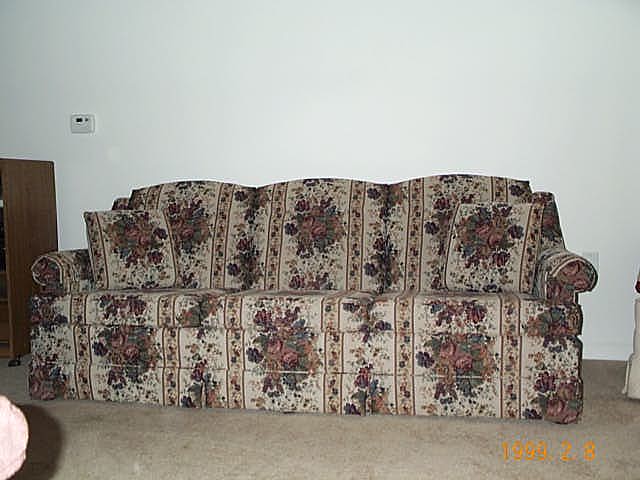The image features an old floral-patterned couch, reminiscent of something found in a grandmother's house. The majority of the couch is a cream color, adorned with vertical, darker cream-colored stripes and large pink roses with green leaves placed in between the stripes. Matching floral-patterned pillows are also visible on the couch. The couch sits on a tan-colored carpet. A small thermostat is mounted on the white wall to the left-hand side above what appears to be a brown wooden dresser or cabinet, only partially visible. The photo, with a date printed in yellow at the bottom right corner suggesting either February 8, 1999, or August 2, 1999, captures this nostalgic scene.